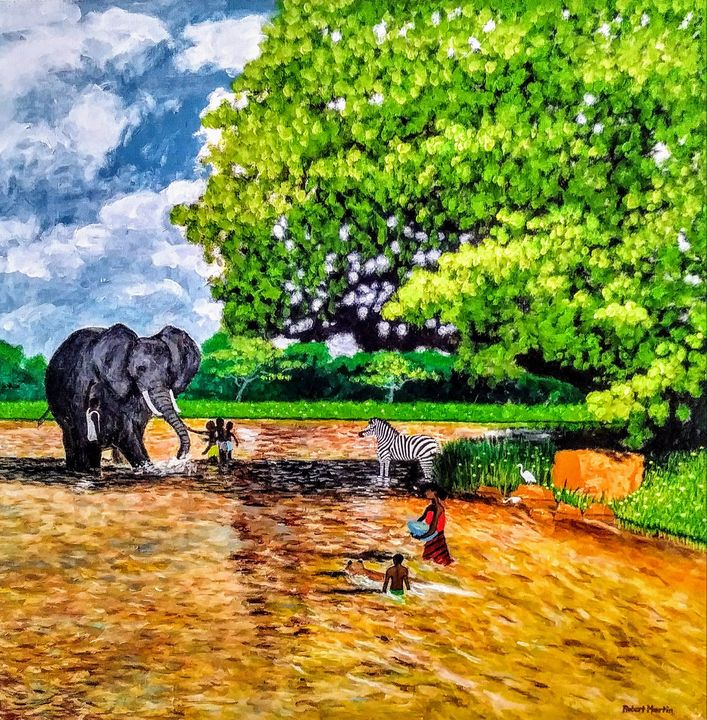This illustration, done in an impressionistic, hand-drawn style with possible pencil or chalk, depicts an idyllic African savanna scene. Dominating the image is a large black elephant with white tusks standing in a wide river, accompanied by a zebra. The river flows through a grassland area with a sprawling green tree on the right, casting shade over the water where the animals and people gather. A group of native people, including some children, are seen petting the elephant, washing clothes, and bathing in the water. In the foreground, one individual holds a basket. To the right side of the river, white swan-like birds can be seen standing on rocks. The background features lush green plains and trees, under a blue sky filled with white clouds.